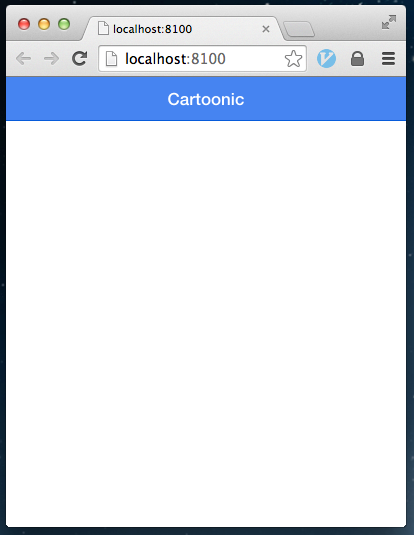Screenshot of a Minimally Displayed Web Page with Errors on a Mac Desktop

This screenshot showcases a portion of an Apple desktop or laptop screen featuring a minimized web browser window, which appears to be experiencing errors or displaying incomplete data. The browser window is cropped to focus solely on its minimized state. It exhibits the distinct Mac user interface, including the iconic red, yellow, and green buttons in the upper left corner of the window, which are used to close, minimize, and maximize the window respectively.

The browser is currently pointing to a local development server, represented by the URL "localhost:8100", which is more akin to an IP address and not a typical public website. The webpage content is sparse, with only a prominent blue banner at the top displaying the text "Cartoonic". The remainder of the page is stark white, highlighting the incomplete or erroneous nature of the displayed data.

Additional elements within the browser interface are also visible, including navigation icons for moving back and forward, refreshing the page, and a star icon for adding to favorites. On the right side of the address bar, there's an icon resembling a widget, a lock icon indicating security settings, and a dropdown menu for more options.

The overall scene captures the essence of a web development or testing environment on a Mac OS, with an emphasis on the minimalistic portrayal of an in-progress web page.